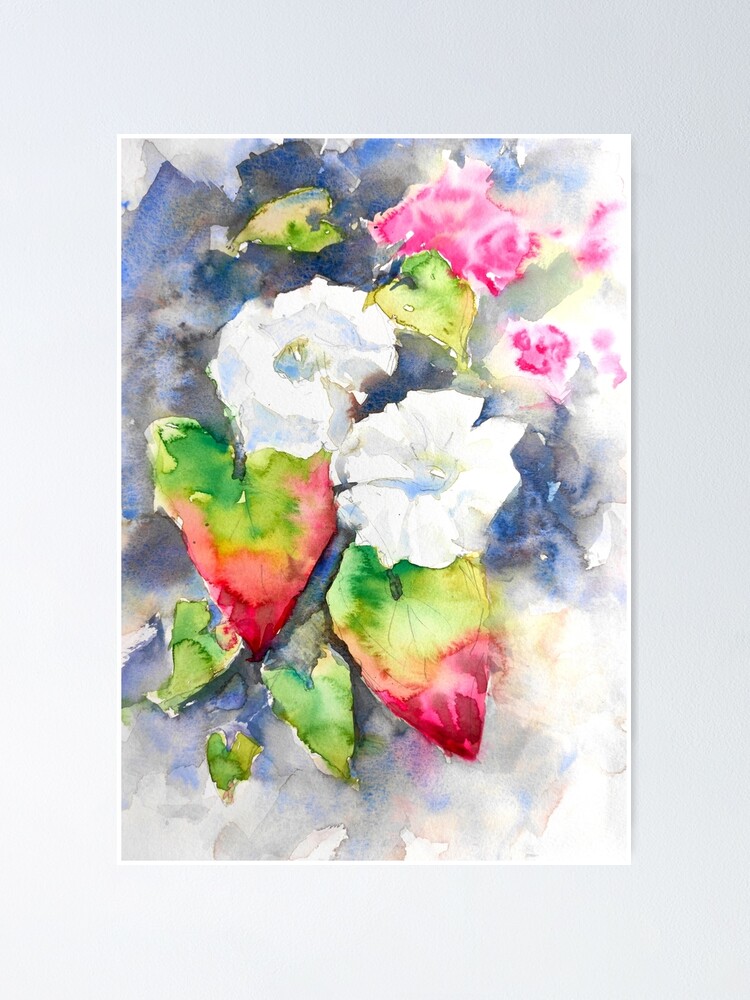This image is a detailed watercolor painting showcased indoors on a light gray wall. A subtle white border frames the vertical artwork, emphasizing its botanical theme. At the heart of the composition are two white flowers with a single row of petals, surrounded by an array of leaves. The leaves display a mix of green shades, some tipped with red or reddish-pink hues. The background is an abstract blend of soft watercolor washes in blue, gray, white, pink, and tan, creating a tranquil and harmonious backdrop. The top right of the painting features a distinct splotch of pink, while the bottom, especially the bottom right, remains the emptiest part of the image, giving a sense of airy space. This precise use of watercolor captures the fluidity and delicate mixing of colors, showcasing the intricate nature of the medium.